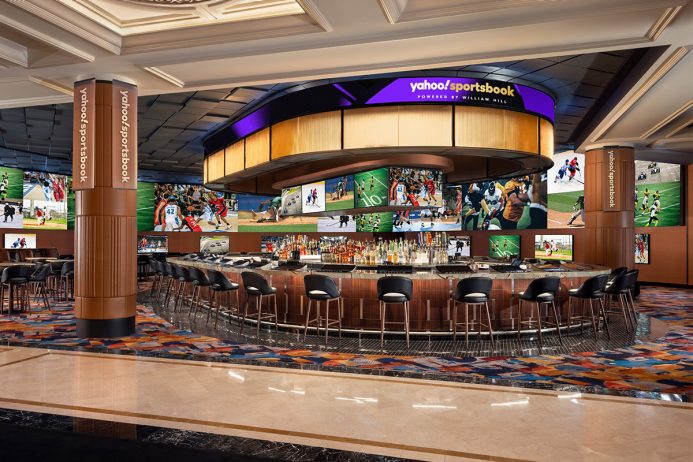This is an image taken inside a sports bar, showcasing a large, semi-circular bar. The bar is surrounded by tall, black high-back stools with wooden legs. Liquor bottles in various colors are neatly stacked and displayed behind the bar. Overhead, the bar has a gold and purple trim ceiling. Numerous television monitors are mounted above the bar and along the walls, displaying various sporting events like hockey, football, basketball, and baseball. Prominently featured on brown banners hanging from two pillars on the left and far right sides of the bar are the words "Yahoo Sportsbook." The room's ceiling alternates between white and black sections, and a vibrant, multi-colored carpet can be seen behind the stools.